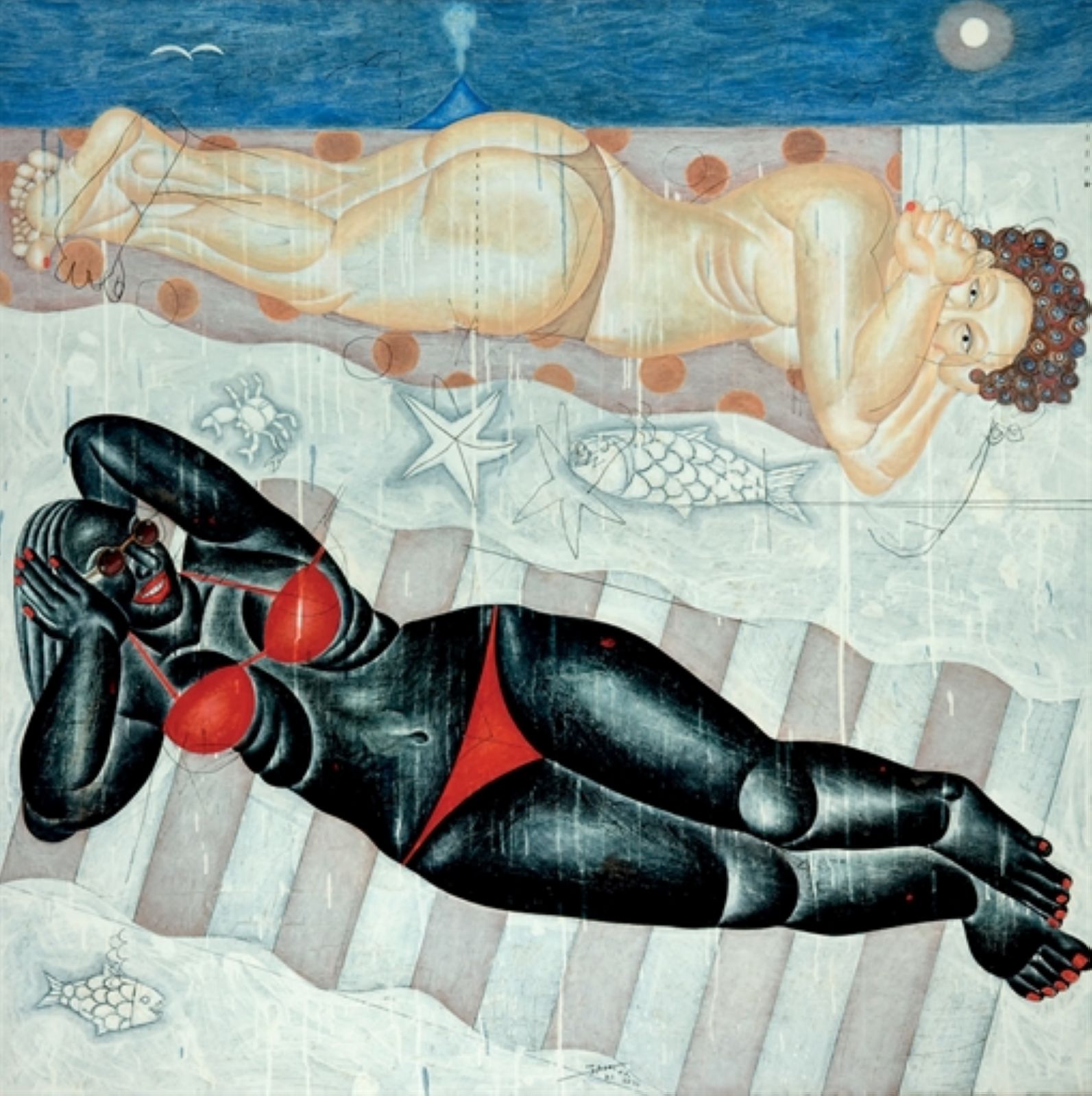This square painting, in an abstract and stylized manner, depicts two women sunbathing near a beach. The top 10% of the image features a narrow blue strip that could represent the sky or ocean, with a white bird-like object on the left and a white dot on the right, possibly a sun. There's a suggestion of a distant volcano emitting smoke. In the foreground, two women lie on purplish-colored rafts in a light bluish-white body of water populated with fish, crabs, and starfish. 

The woman on top has a light beige skin tone, defined muscles, and is wearing a brown G-string thong. She is laying on her stomach, slightly turned to her side, with her arms covering her breasts and her hand near her mouth. She has curly brown hair and is positioned horizontally on an orange and purple towel. 

Below her, the second woman has skin that is a striking blackish-blue color, not a naturalistic brown, and she is wearing a red bikini. She has matching red accessories including lipstick, nails, and circular sunglasses. She is laying on her back, smiling up at the viewer on a striped towel with purplish-gray and whitish-blue hues. The composition of the image, with its offbeat colors and flattened perspective, exudes a unique and surreal atmosphere.